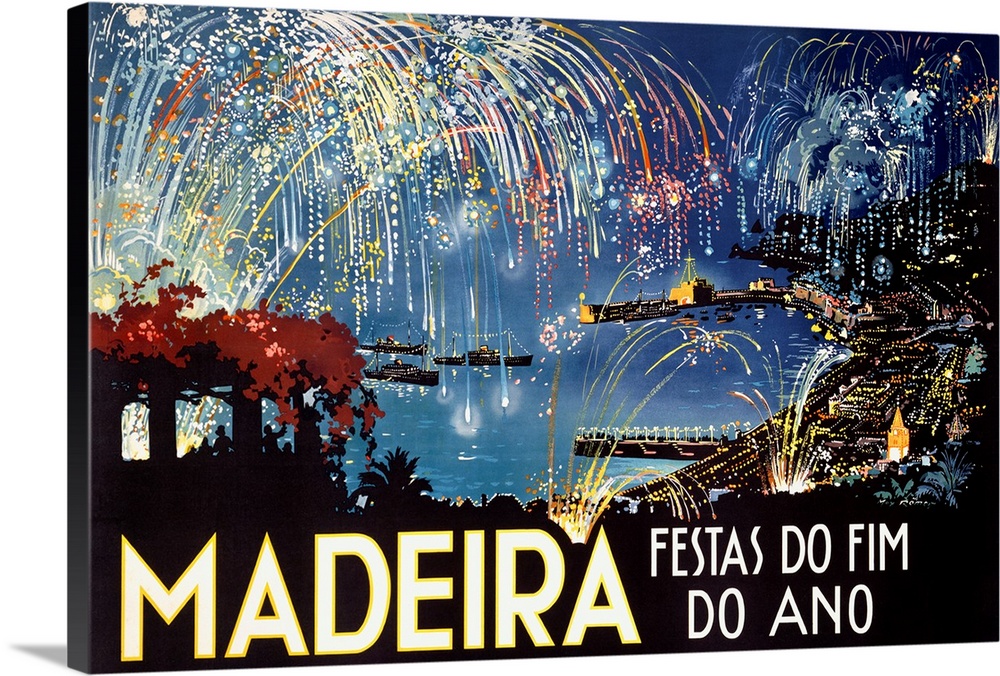This vibrant and colorful image, likely a print on canvas or an art piece, depicts a lively firework show over the coastal city of Madeira during the nighttime. The scene captures a festive atmosphere, possibly memorializing an event named "Madeira Fiestas do Femme do Ano," which is written in tall, capital white letters at the bottom in a foreign language, resembling Spanish. In the foreground, a family of dark silhouettes stands under a roofed structure adorned with red flowers, pointing and cheering at the dazzling display. A cluster of trees with red leaves further enhances the scene. The cityscape is beautifully illuminated with yellow lights from various buildings, boardwalks, and piers, casting a warm glow across the waters below. Fireworks of vibrant yellows, blues, whites, reds, and oranges burst from multiple locations in the sky, reflecting in the water where boats are docked along a pier. This picturesque, postcard-like image captures the essence of a joyous celebration by the sea.